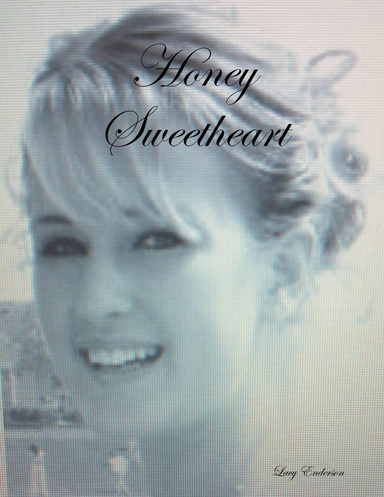The photograph appears to capture a striking portrait of a young Caucasian woman in a side profile. Her hair, which is light in color and pulled up in the back with long bangs framing her eyes, suggests a formal occasion, possibly a wedding. She gazes directly at the camera with a joyful smile, her face framed prominently in the center of the image. This black and white photo reveals subtle hints of gray and off-blue tones, adding to its vintage feel. The detailed pixels suggest it may have been photographed from a computer screen. The woman wears noticeable mascara, accentuating her eyes. In elegant black cursive script, the words "Honey Sweetheart" are placed near her forehead, and a barely legible signature, possibly "Lacey Anderson," is inscribed in the bottom right corner. The background features distant figures, adding depth to the intimate portrait.